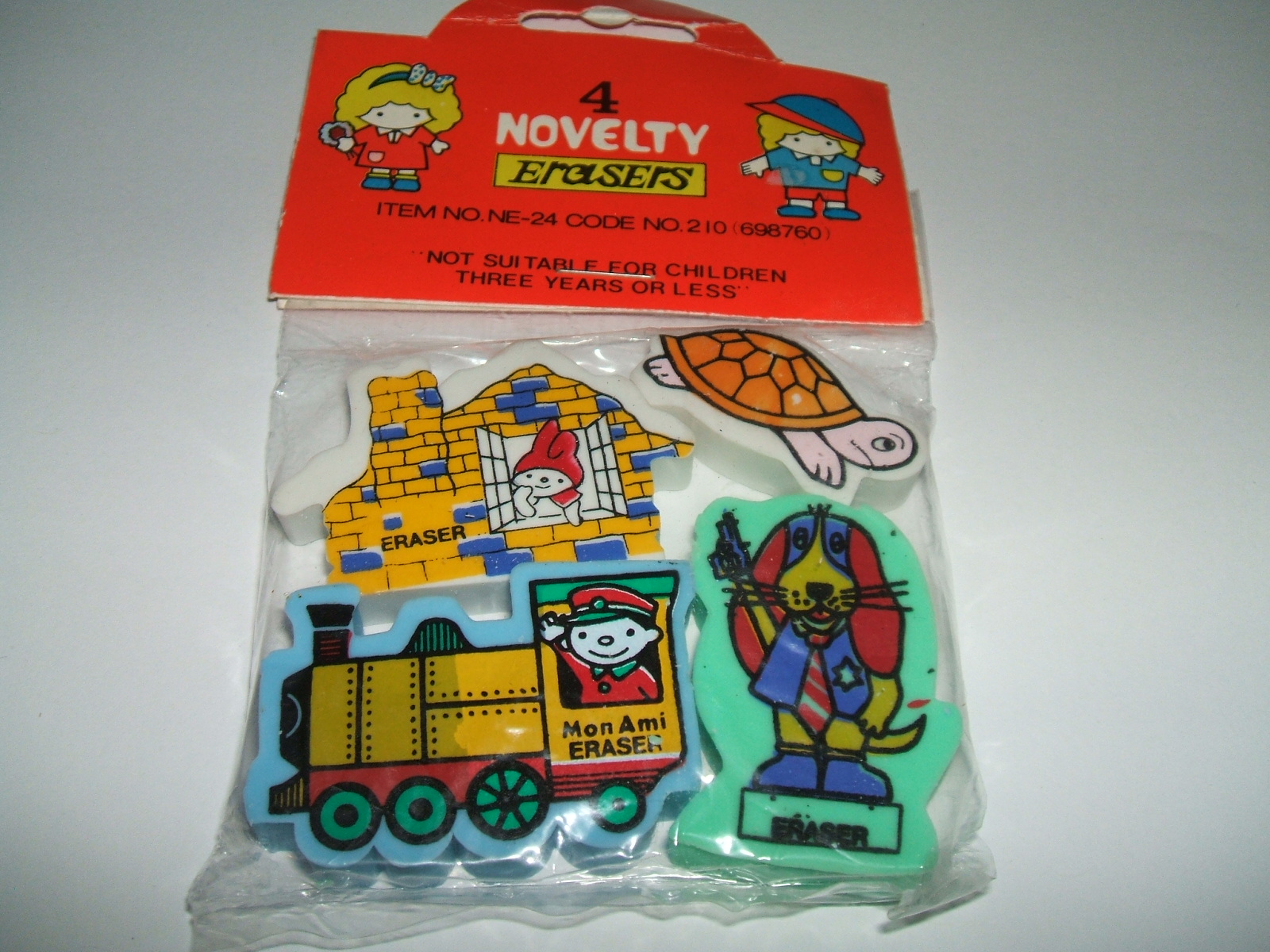This image features a colorful set of four novelty children's erasers, still sealed within their original packaging. The erasers are housed in a clear plastic bag, which is stapled shut at the top with a piece of vibrant red cardboard. This header card, designed to catch the eye of potential buyers, displays a cartoon illustration of a boy and a girl, both with blonde hair. The text on the cardboard prominently reads "Four Novelty Erasers" and includes an item number along with a warning that the product is not suitable for children aged three years or less. 

Inside the clear bag, the erasers are vividly detailed and whimsical. The first eraser depicts a bunny looking out of a window, seemingly from a yellow and blue brick house, while wearing a red hood. The second eraser portrays a dog, possibly a beagle with long ears, holding what looks like a pink sword or ribbon. The third eraser features a smiling train conductor. Finally, the fourth eraser is shaped like a frowning turtle with a white body and an orange shell. The entire package rests on a white table, emphasizing the nostalgic charm of this unopened, kid-friendly product designed for impulse buys at store checkouts.